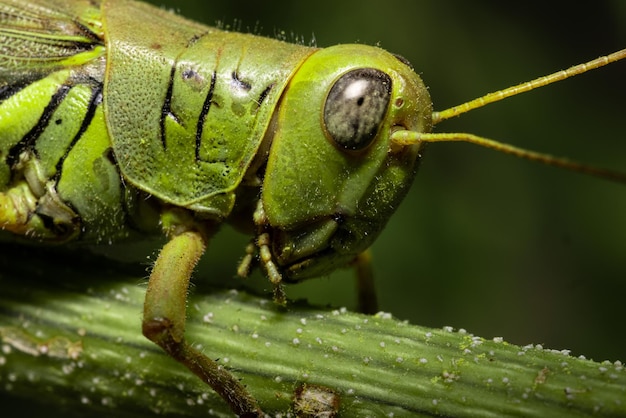This is an extremely close-up image of a green grasshopper, captured in exquisite detail. The background is a blurry blend of green hues, causing the grasshopper to stand out prominently. The insect is perched on a green, tubular stalk adorned with tiny white dots. The grasshopper's head, which is oval-shaped and green, features a large, slightly cloudy, black eye with hints of gray. Its two thin, green antennae extend outward. 

The creature is in profile facing to the right, allowing a clear view of its body from just below the wings to the head. A striking section, resembling a red or green cape or jacket, covers the top part of its body and joins seamlessly with the bright green lower body, which is embellished with black lines. One of its legs can be seen gripping the stalk, with tiny, clear hairs dotting the area around the leg and the rest of its body. The combination of these intricate features and the blurred backdrop creates a vivid and detailed portrait of the grasshopper.